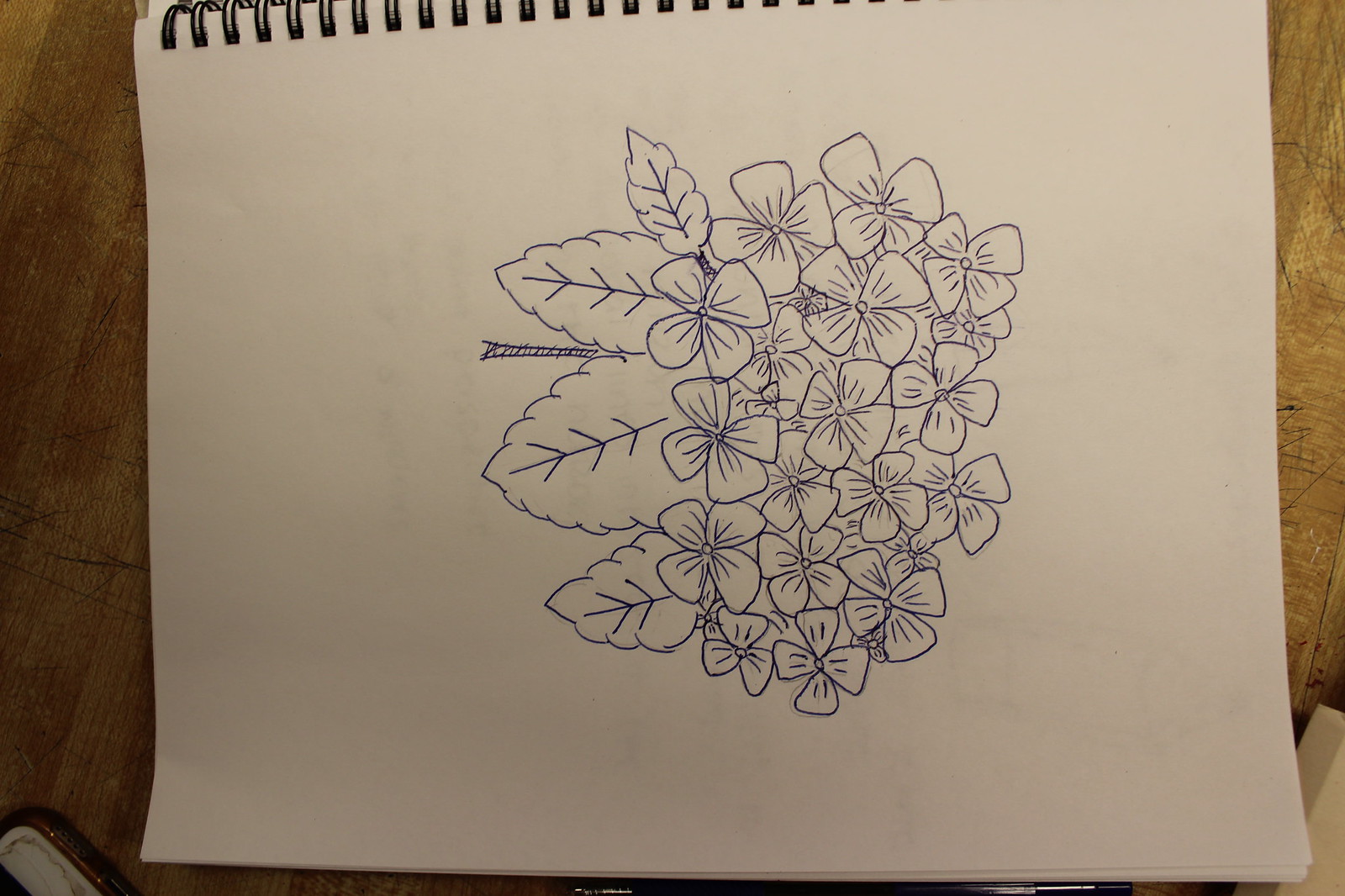The image showcases a sketchbook positioned on its side, its metal coil binding distinctly visible at the top. Inside, a large, blank sheet of paper serves as the canvas for a blue pen drawing. The artwork features a cluster of small, delicate flowers and several sizable leaves. The flowers, concentrated either at the top or bottom of the drawing, are balanced by four prominent leaves on the opposite side. Despite the monochrome blue, the intricacy of the pen strokes gives life to the uncolored flora. The sketchbook rests on a wooden table, apparent by the visible scratches and wear, suggesting frequent use. In the bottom right and left corners of the image, two indistinct objects can be seen on the table, adding depth to the scene without detracting from the central focus of the sketch.